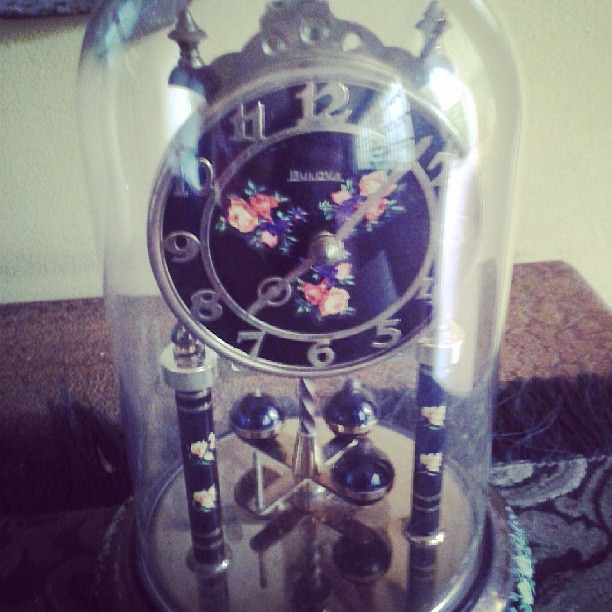This is a slightly grainy photograph of an ornate Bulova clock encased in a clear glass dome, set against a white wall. The clock face, painted in navy blue and adorned with delicate red, white, pink, and blue-green floral designs at the center where the hour and minute hands meet, features Arabic numerals. The clock is positioned on a base supported by four pillars, also decorated with flowers in soft yellow hues, and these pillars rise from a reflective, round surface. Below the clock, a complex pendulum mechanism with arms that extend outward, each holding four black shiny balls, suggests a delicate swaying motion. Despite the slight blur and reflections on the glass, creating some uncertainty about the exact time displayed, the detailed craftsmanship of the clock is evident. The base beneath the clock appears to rest on a material that could be fabric or patterned cloth, adding a subtle texture to the background.